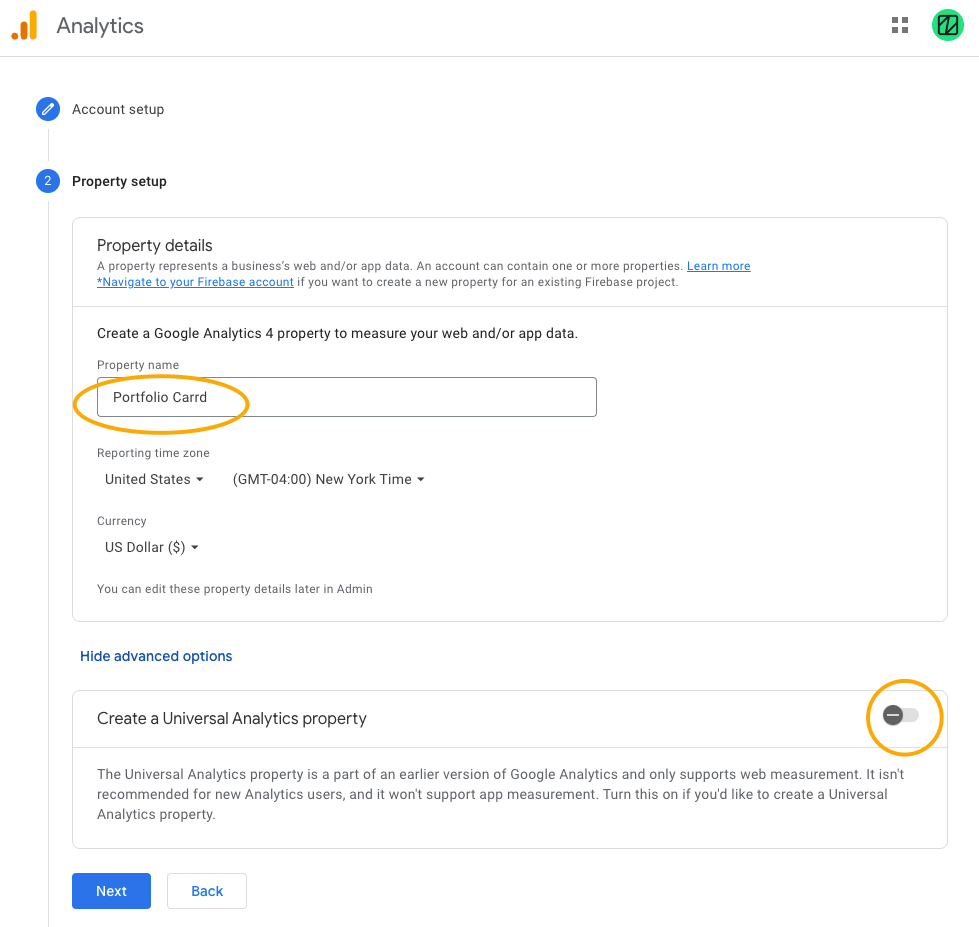Screenshot Description: 

The screenshot displays the back end of Google Analytics during the account setup process. The top-left corner of the interface showcases the Google Analytics logo accompanied by the label "Analytics." Directly below the logo is a menu item labeled "Account Setup," featuring an adjacent edit button. Underneath this, another menu item labeled "Property Setup" is highlighted, indicating that it has been selected.

The main section of the screenshot focuses on the "Property Setup" settings. The interface prompts the user to create a Google Analytics 4 property to measure web and/or app data. It instructs users to input a property name, which is specified as "Portfolio Card" in this example. To draw attention, the property name "Portfolio Card" is circled in the screenshot. Further down, fields for "Reporting Time Zone" and "Currency" settings are visible, followed by expandable "Advanced Options."

One notable setting at the bottom of the screen is a toggle option for "Create a Universal Analytics property," allowing users to enable or disable it as per their requirements.